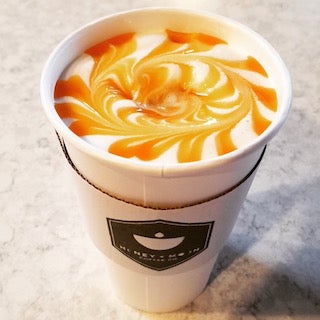The image features an elegantly placed disposable white coffee cup with a matching white sleeve adorned with a black shield-shaped logo, showcasing a distinctive white dot and half-moon design. The coffee inside exhibits an intricate swirl of vanilla and caramel, creating a mesmerizing pattern that suggests careful craftsmanship. This detailed design of white and orange hues mirrors the counter-clockwise motion, likened to the appearance of a hypnotic or candy-cane-inspired motif. Despite the ornate topping, which resembles foam or whipped cream embellished with copious caramel, no steam is visible, indicating the drink might be cold. The cup rests on a sophisticated white and gray marble countertop, and strong lighting enhances the scene, casting shadows to the right and highlighting every aspect of the meticulously swirled beverage.